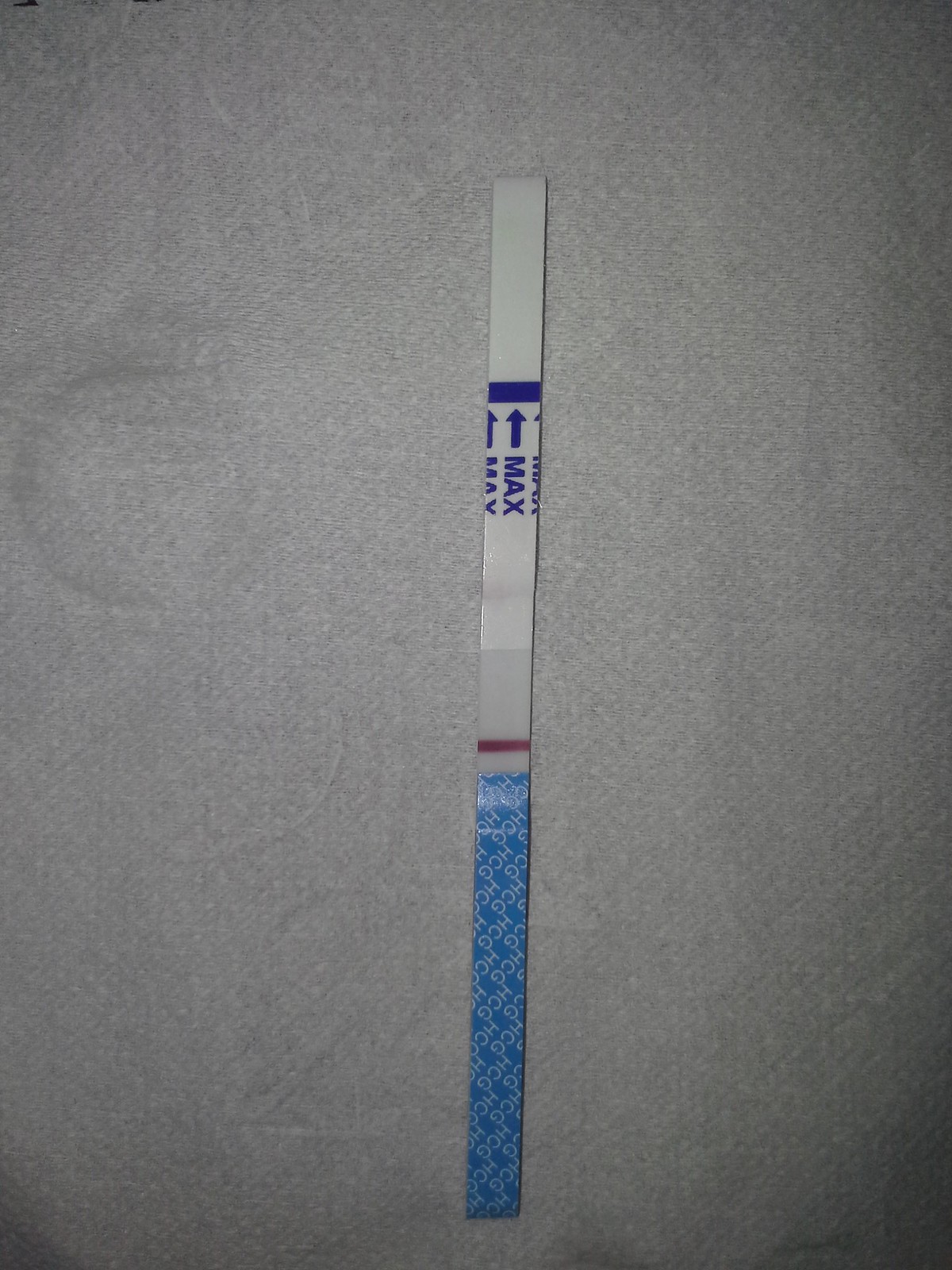A long testing strip is vertically positioned on what appears to be a quilted paper towel, reminiscent of cloth in its texture and softness. The test strip is divided into distinct sections. The top half is predominantly white, featuring a prominent horizontal blue stripe. Above the stripe, a bluish-purple arrow points upward with the word "Max" labeled just at the stripe's edge. Approximately midway down the strip, there's a faint red line, slightly blurred at the edges. The lower half of the strip transitions to a blue background, decorated with a white, diagonally-repeating "HGC" pattern.